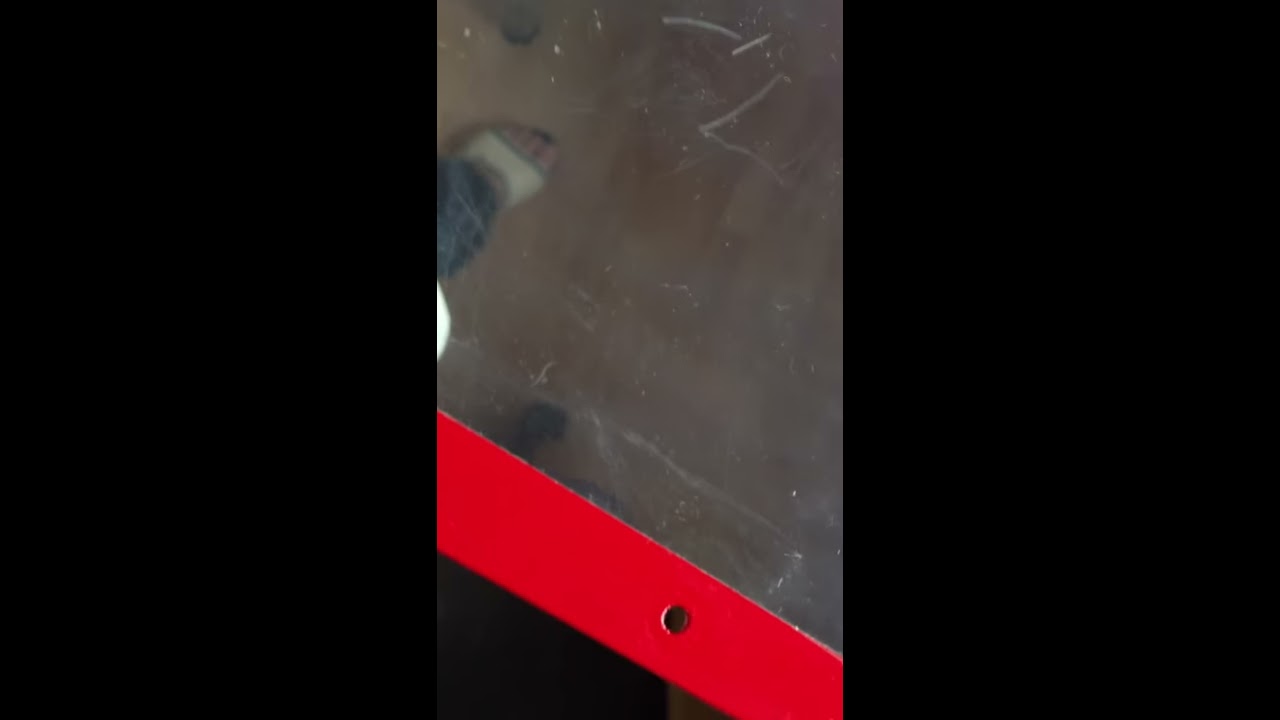The image consists of three vertically divided, equal-sized rectangles: with the left and right rectangles completely black. The central rectangle reveals an overhead view of a brown, slightly scratched cement floor. Dominating the image is a prominent, bright red bar slanting from the top left to the bottom right, featuring a single circular hole on the lower right of the bar. At the top of the central section, a partially visible left foot, clad in light gray socks with black and gray accents and a white sandal exposing the toes, is seen touching the ground. Notably, a white scratch resembling the number "2" is in the upper right corner of the floor, adding an intriguing detail to the otherwise minimalistic scene.